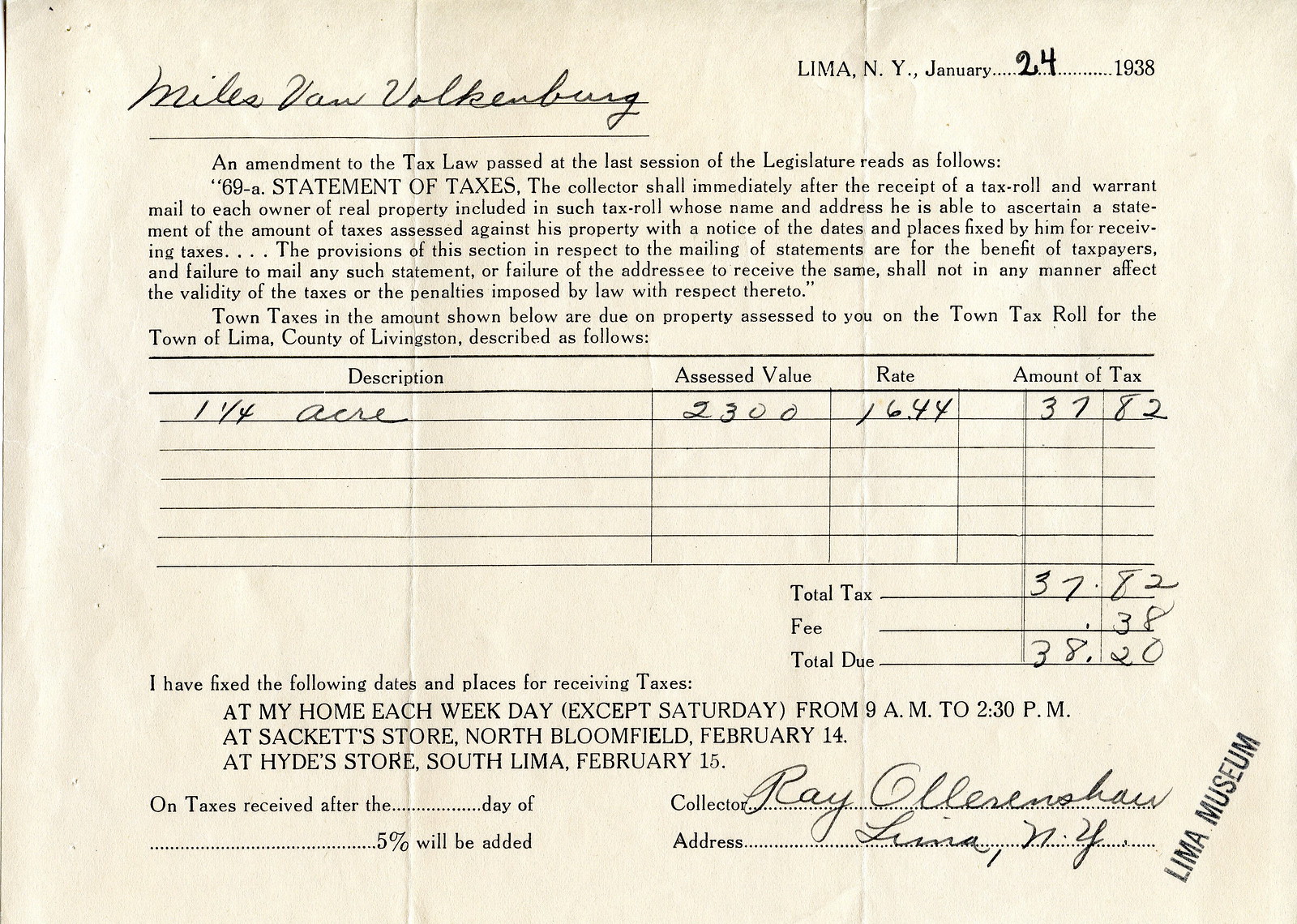The image depicts an old, weathered tax bill set horizontally. At the top left corner, there is a cursive script reading "Miles Van Valkenburg," which is underlined. In the top right corner, the document specifies "Lima, New York, January 24, 1983." Following this, a typed paragraph includes an amendment to the tax law: "An amendment to the tax law passed at the last session of the legislature reads as follows: The collector shall immediately after the receipt of a tax roll and warrant mail to each owner of real property included in such tax roll a statement of the amount of taxes against their property." Below this paragraph lies a small grid organized into several columns with labels: "Description" (indicating "one and a fourth acre"), "Assessed Value" (noted as 2300), "Rate" (17.44), and "Amount of Tax" (3782). Further below, there is a section labeled "Total Tax" with handwritten figures: 3782 for the total tax, a fee of .38, and a "Total Due" of 38.20. At the bottom right, the collector's name, "Ray Allen," is handwritten in cursive, followed by the address "Lima, New York."